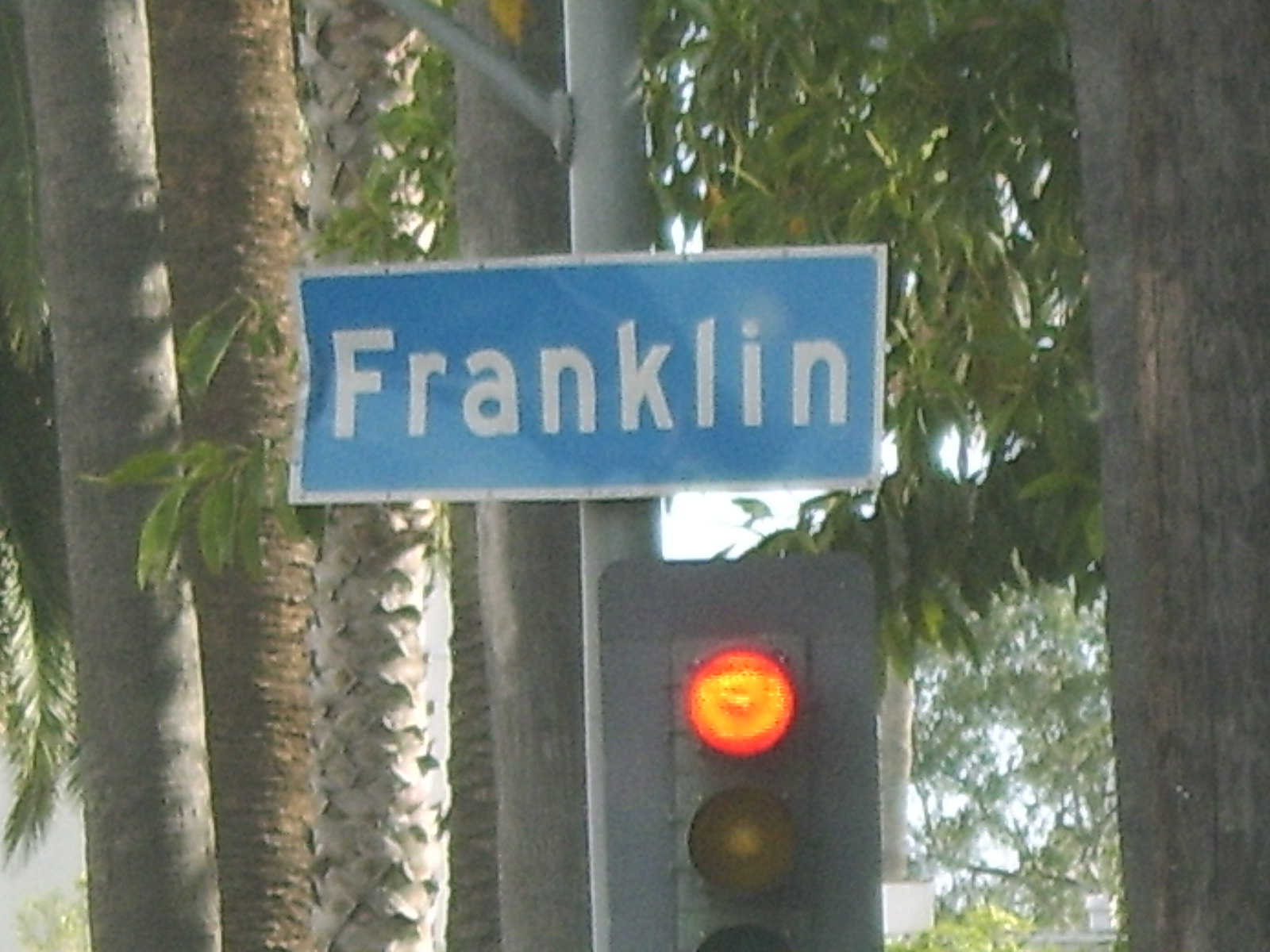The image depicts an outdoor scene with a prominent blue street sign in the center that reads "Franklin" in white text. The sign is mounted on a silver pole that extends vertically through the image. Just below the sign is a traffic light featuring a lit red light, with spaces for yellow and green lights below it. To the right of the pole stands a large tree with deep green leaves interspersed with light shining through, revealing a few bare branches and some leaves hanging down. The background showcases a row of trees in shades of brown, gray, and white, including a birch tree, contrasting with patches of blue sky and white clouds visible through the foliage. The overall composition combines structured elements like the street sign and traffic light with the natural, textured environment of the trees and leaves.